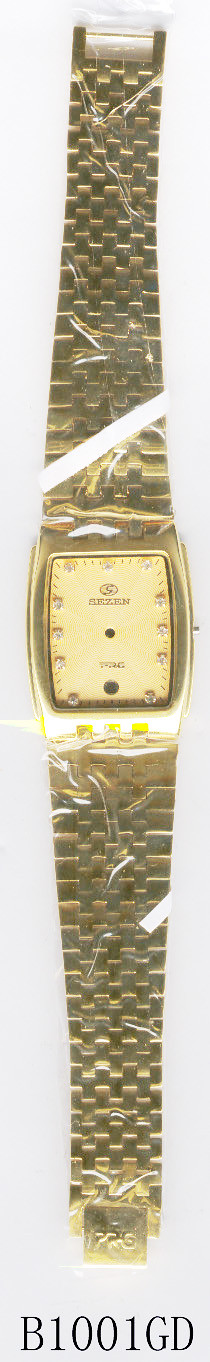The image features a sophisticated gold watch, prominently displaying the brand name "GEZEN" on its elegant rectangular clock face. The watch is carefully positioned flat within a clear plastic bag, suggesting it's either brand new or part of an advertisement showcase. Instead of traditional numbers, the watch face is adorned with small, refined dots marking the hours. The strap is composed of classic gold chain links, reminiscent of timeless designs often favored by older generations. Below the watch, printed on the plastic bag or on a label, is a distinct identification code: "B1001GD" in bold, capital letters.